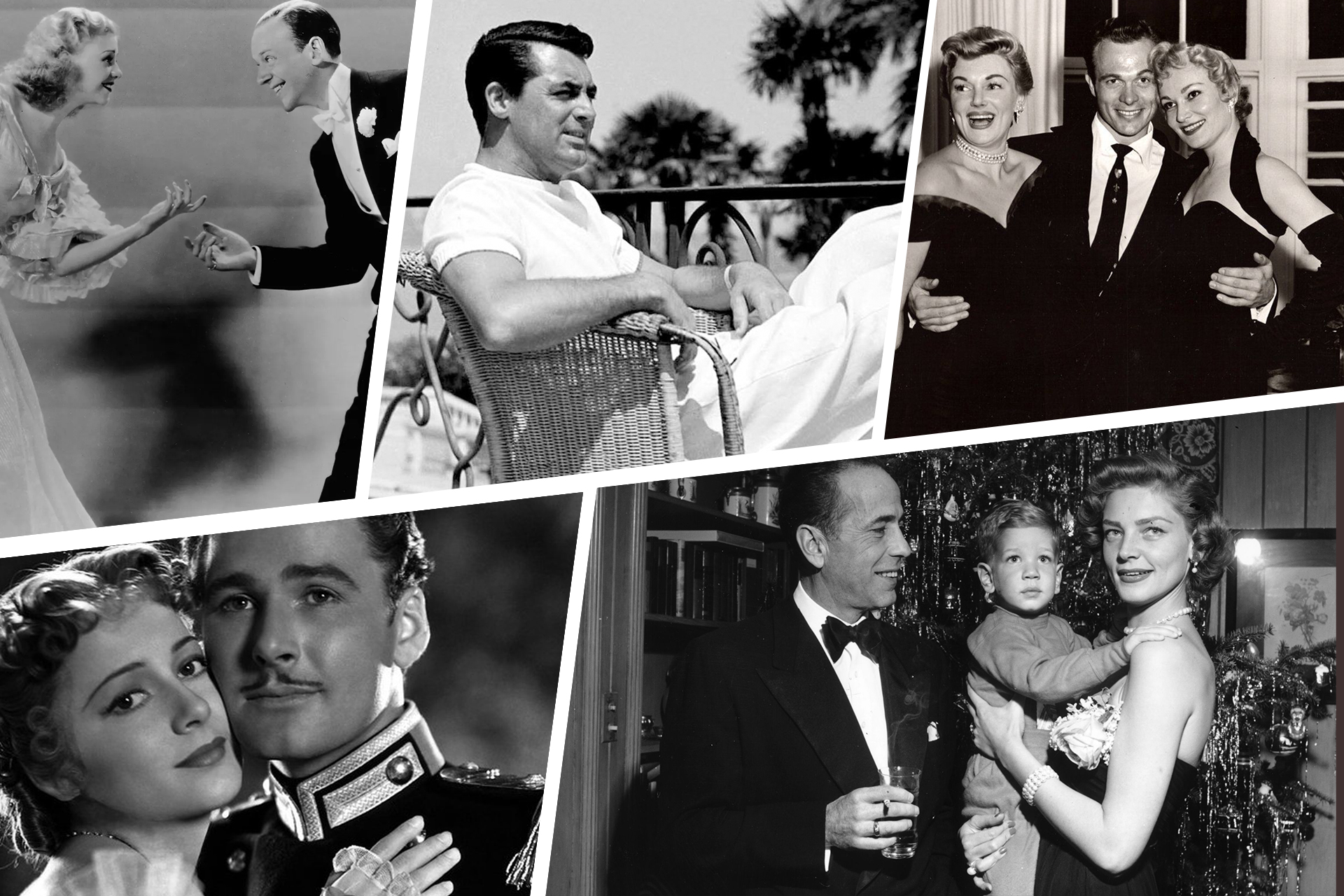This photo collage consists of five black-and-white images featuring movie stars from the early 20th century, likely from the 1930s to the 1950s. 

The top left image depicts a man and a woman about to dance; the man is dressed in a formal suit while the woman wears a dress with her hair styled in curls. 

In the top center, there's a casual-looking man sitting in a wicker chair outdoors, possibly in a tropical location. 

To the right, in the top right panel, a man in a suit is posing with two women in black dresses, adding a touch of glamour to the scene. 

In the bottom left image, a close-up shows a man and a woman in what appears to be a uniform, their faces close together in an intimate embrace. 

The bottom right image displays a family scene: a man holding a drink and cigarette looks at a woman who is holding a small boy. They appear to be in a living room with paneled walls and a bookcase, possibly at a party.